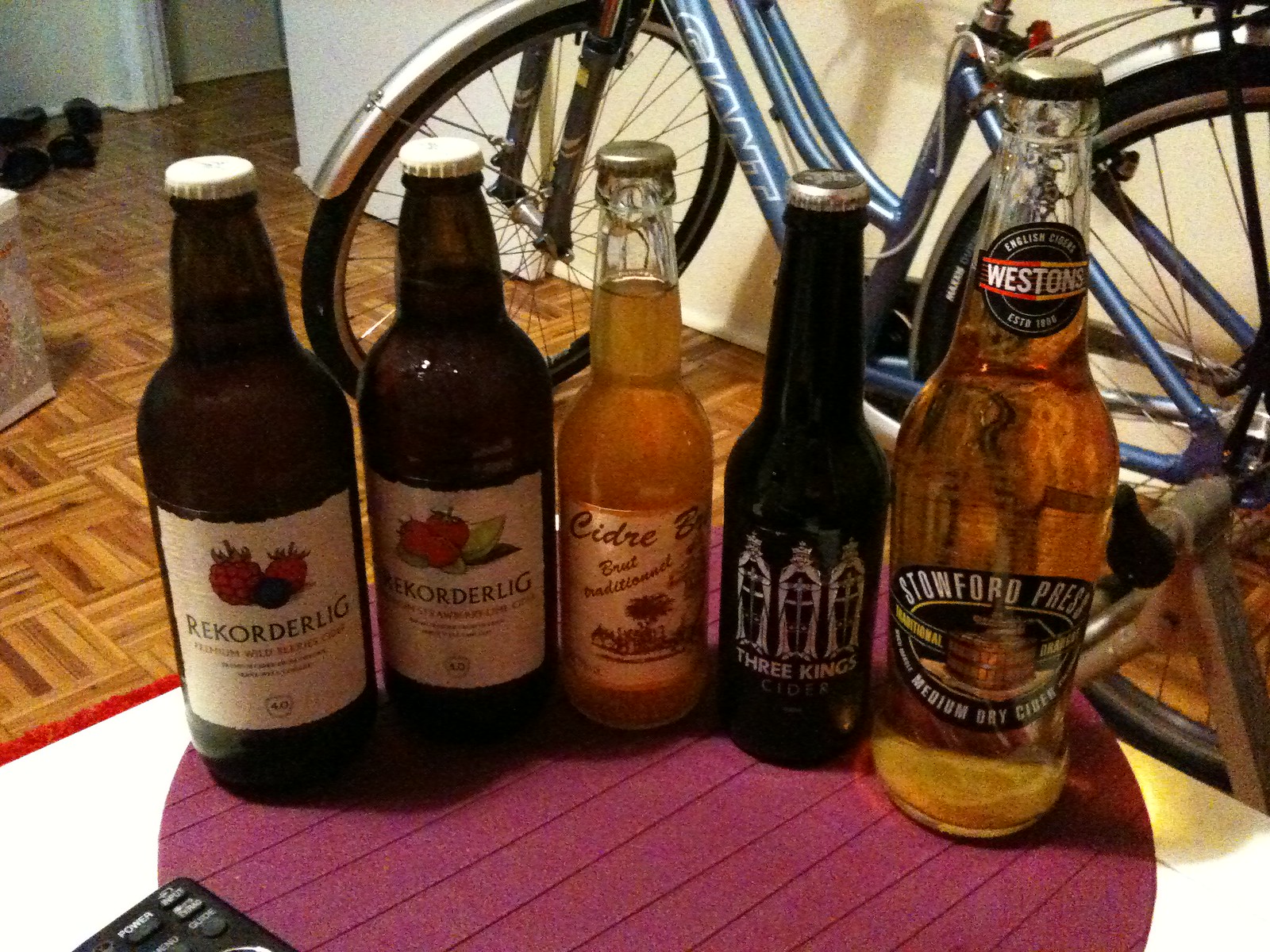This image depicts a small table adorned with a circular maroon tablecloth featuring vertical and horizontal lines, set against a backdrop of a light brown wooden floor with a square tile design. On the tablecloth, five bottles of cider are neatly lined up, each with their labels clearly visible. The first two are short brown beer bottles with white caps, both branded "Rekorderlig," displaying labels with fruit illustrations—one with raspberries and blueberries, the other with a green apple slice and strawberries. The third bottle is thinner with a light gold liquid inside and a label that reads "Cidre," although the full text is obscured by the bottle's curve, accompanied by tree illustrations. The fourth bottle is a dark, almost black bottle labeled "Three Kings Cider," featuring white king-like figures on a black background. The last bottle is a taller one with a gold liquid inside, a silver cap, and dual labels—a black circle on the neck reading "Weston" and a black oval on the front that says "Stoufford Press, Medium Dry Cider." Behind the table, a blue bike leans against a white wall, a pair of black shoes is visible on the floor, and a remote control peeks out from under the table.